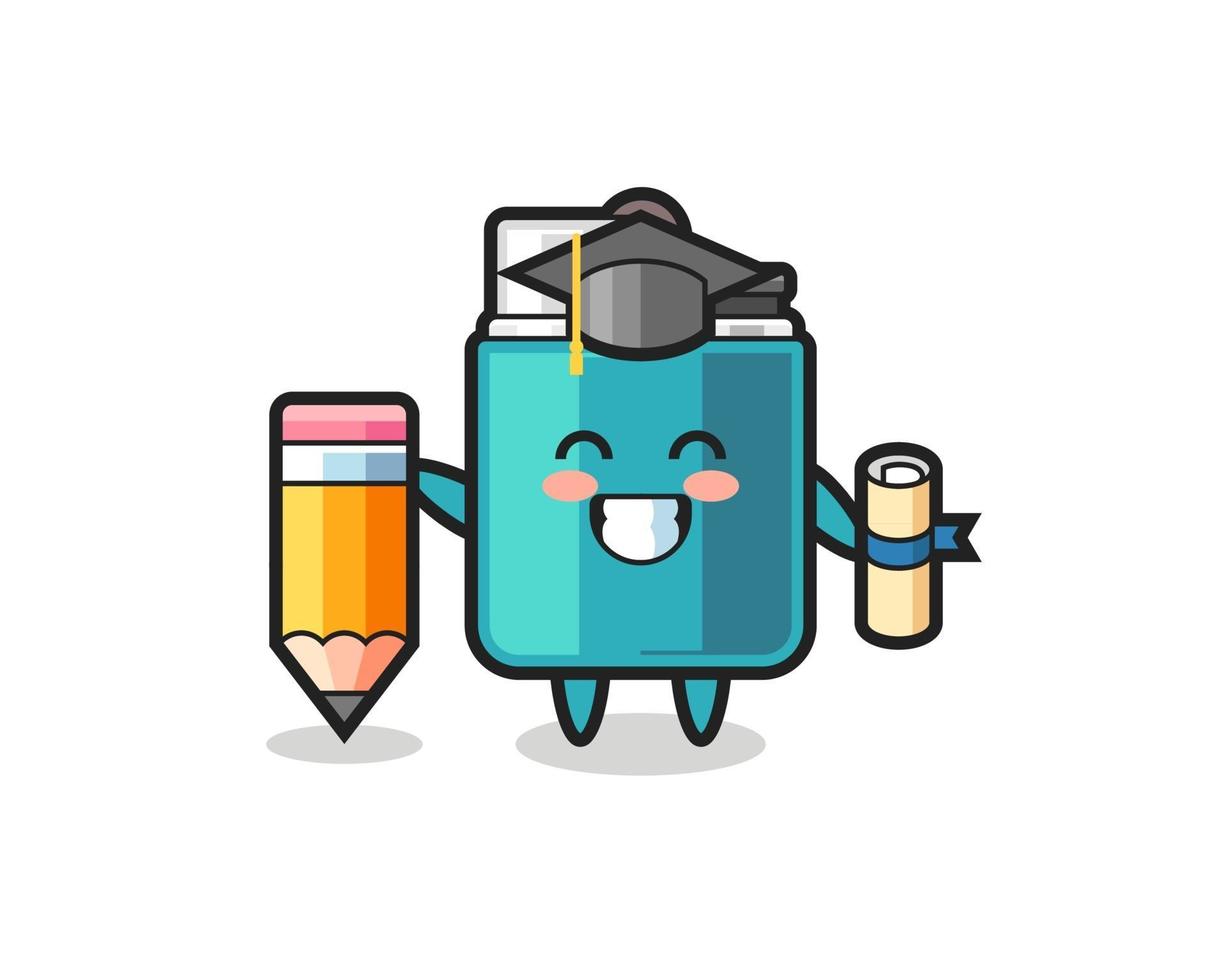This digital cartoon image features a cheerful blue square character with legs, arms, and no nose. It has expressive blue eyes, prominent white teeth, and rosy pink cheeks. On its head, it wears a black graduation cap adorned with a yellow tassel, signifying a celebratory occasion. In its left hand, the character proudly holds a diploma, wrapped in a blue ribbon, while its right hand grasps an oversized yellow pencil that extends almost to the character's head. The background is a solid white, making the colorful cartoon figure stand out vividly. The character's joyful expression and academic accessories give it a lively and humorous appearance.